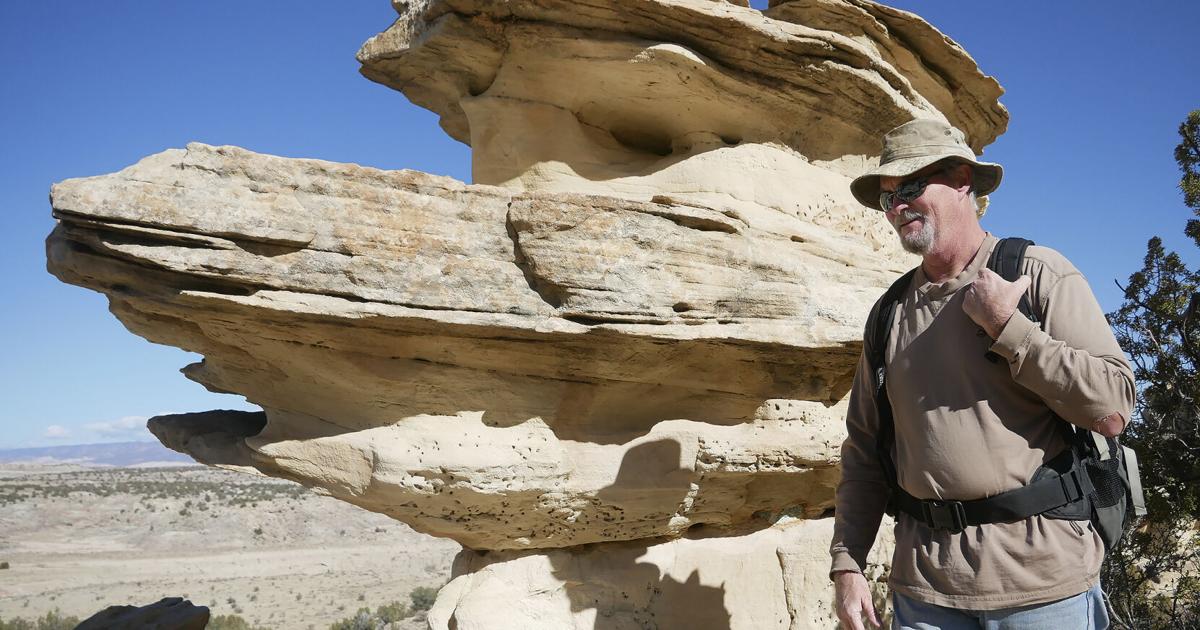A man of Caucasian descent, slightly facing the left side, is standing in front of a large, natural rock formation that appears to be a collection of five rocks melded together. The stone structure has numerous ridges and holes, reminiscent of erosion from flowing water. The man is decked out in a light brown boonie hat, black sunglasses, and a beige or tan long-sleeved shirt, which seems to have holes at the elbows. He sports a gray mustache and goatee and is smiling subtly. A black hiking backpack is strapped around his waist, with the shoulder straps visible; he holds the left strap with his bent left arm, while his right arm hangs by his side. His blue jeans complete the outfit. The backdrop includes a clear blue sky with low clouds and a distant view of water, surrounded by trees and dirt terrain, suggesting a high elevation. This photo captures him during a sunny day, possibly after a hike, as he poses near the impressive rock formation.